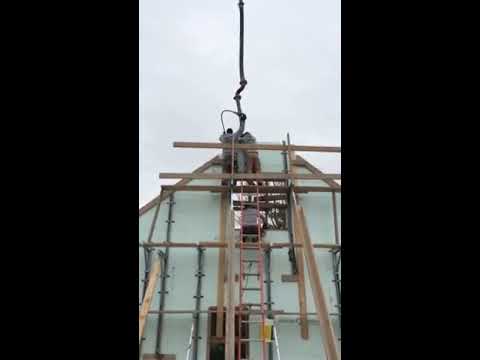The image is a vertical photograph with black borders on the left and right, set against a light grayish blue sky, possibly overcast. The scene depicts an outdoor construction site in daytime, showing a building still in the process of being constructed. The unfinished exterior is a light mint green and predominantly covered with a mix of metal and wooden scaffolding. In the center, there's a ladder leading up to two workers at the top part of the scaffolding. They appear to be handling a black pipe, possibly a drainage pipe. The workers, dressed in gray outfits, seem unprofessional and the environment appears chilly. The structure features a triangular roof though parts are visibly incomplete, a door frame at the bottom, and an area that could be intended for a window.